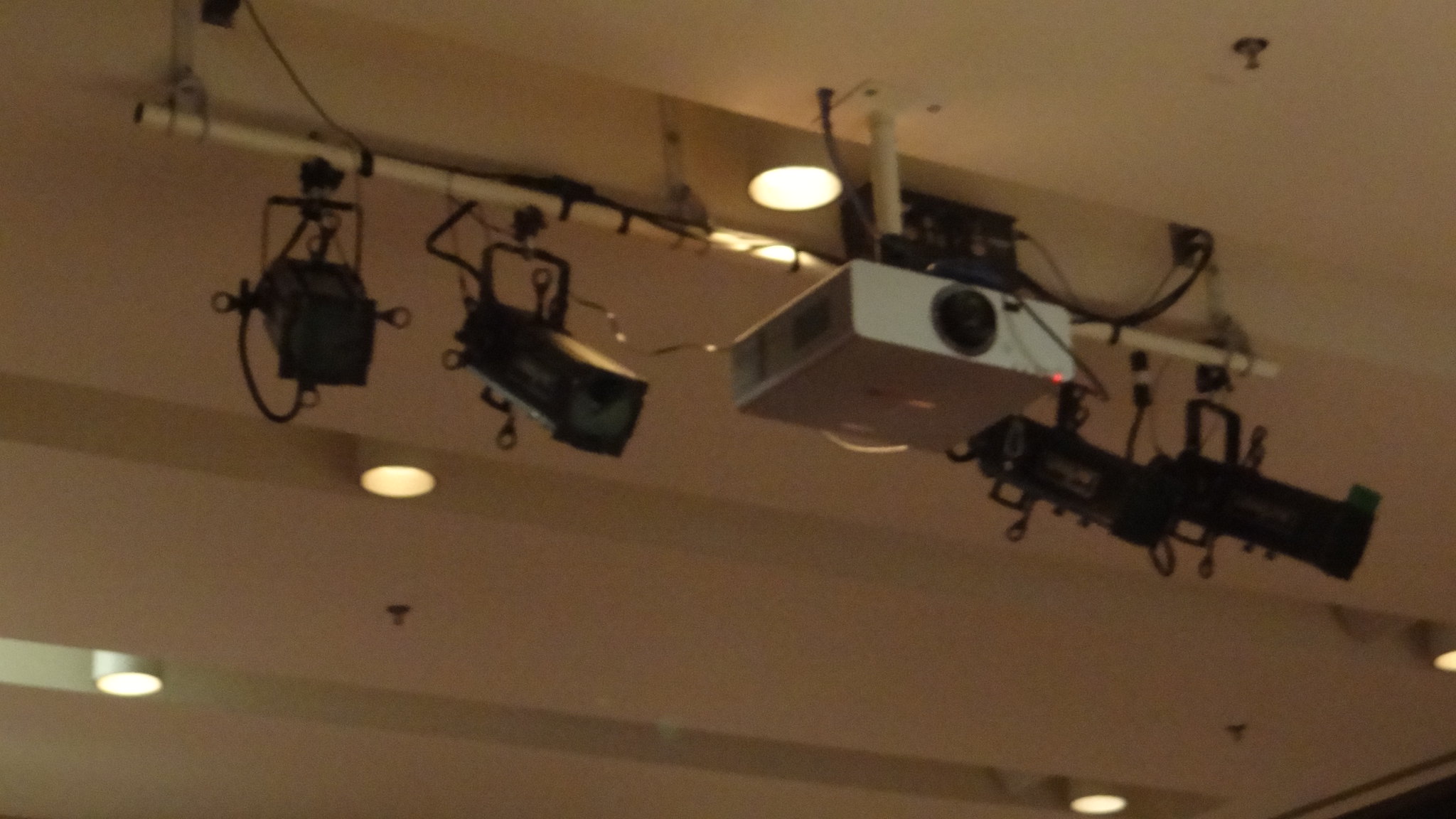This indoor color image reveals an auditorium ceiling from a slightly angled, upward perspective. Dominating the upper half of the image is a white bar supporting essential audiovisual equipment. At the center of the bar hangs a white projector, identifiable by its black lens covering. Flanking the projector are four black stage lights, angled diagonally downward toward the lower right corner of the image. The ceiling is white with five recessed lights and features a complex, non-flat structure with angled sections. Additionally, three sprinkler heads are visible, projecting from the ceiling. The image is dimly lit and out of focus, capturing the typical setup of equipment essential for stage presentations in an auditorium.